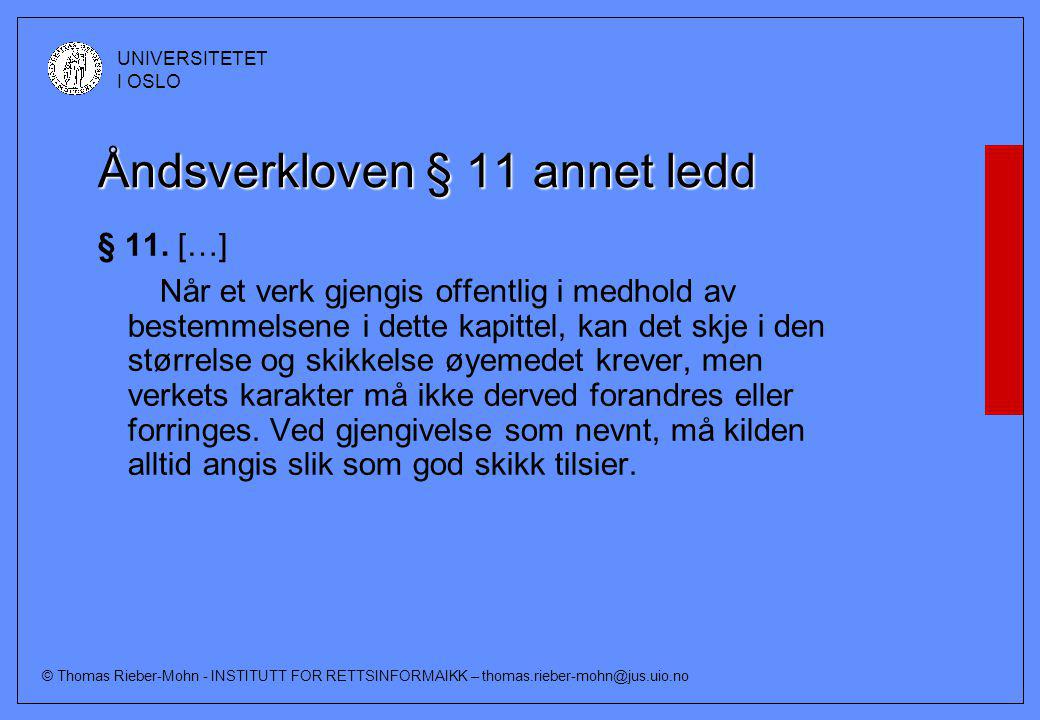This image is a blue rectangular PowerPoint slide bordered by a thin black pinstripe. Along the right edge, there is a distinctive red vertical bar. In the top left corner, a round, indistinct black-and-white logo is visible alongside the text "Universitet i Oslo." The slide's title, featuring the word "Andsverkloven," is prominently displayed in larger, black text with white edging, followed by a paragraph in smaller, bold black text written in a foreign language, possibly Norwegian. Towards the bottom left, the text reads "© Thomas Reber Moen, Institute for Rettsinformatikk," with an email address "Thomas.Reber-Mohn@jus.uio.no." The overall design is minimalistic, primarily text-focused, and seems to emphasize academic content.